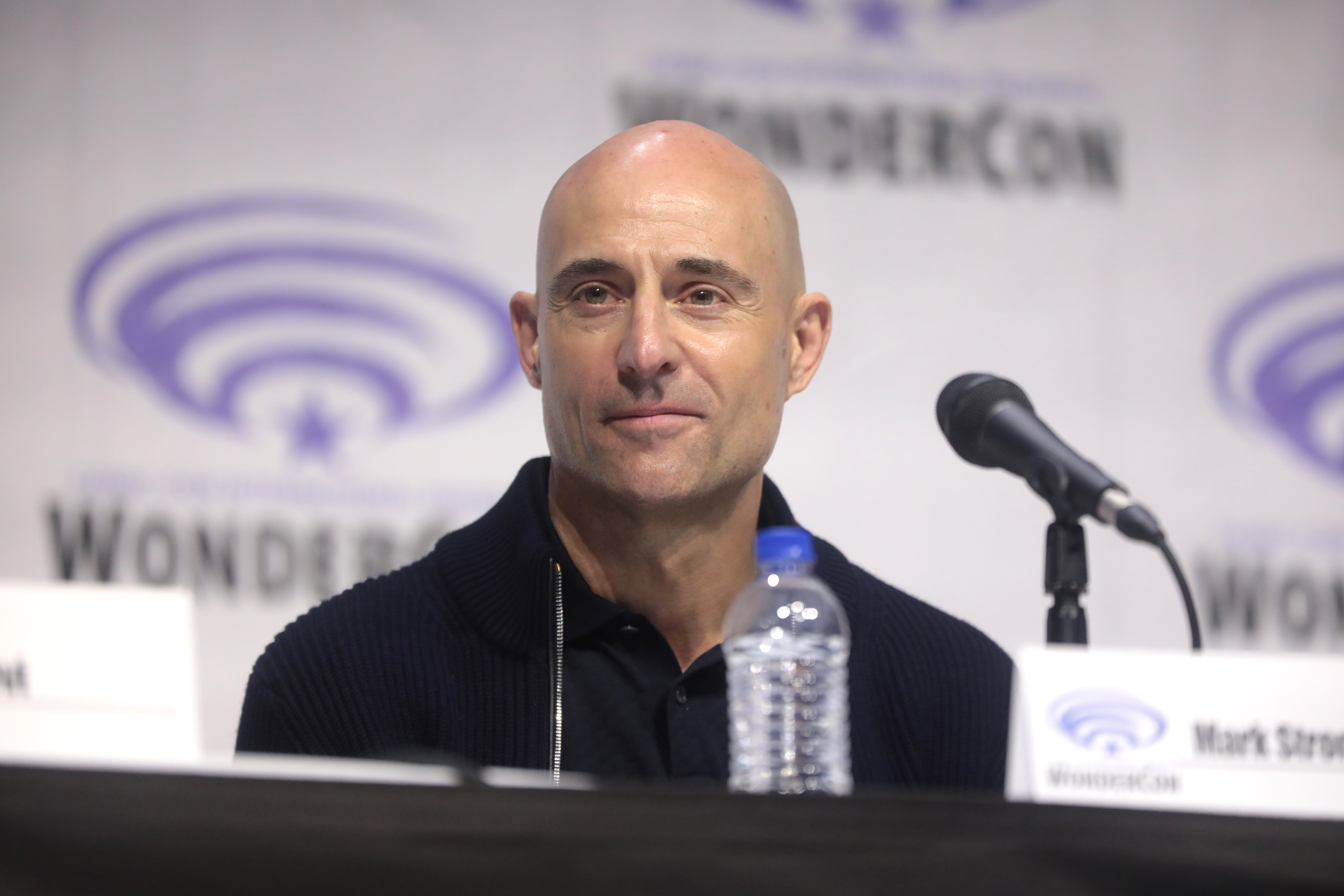In the photo, a man named Mark Strong is seated at a podium, with only his head and shoulders visible. He has dark eyebrows and a bald, shiny head, wearing a black button-up shirt with a matching black collar. A black microphone is propped up to his right for him to speak into, and a clear plastic water bottle with a blue lid sits in front of him on the table. There is also a white name tag in front of him with a blue logo. The background features a blurred white wall with the logo and writing of WonderCon, including a blue star with swirls above it. Mark Strong appears to be smirking slightly and looking to his right.